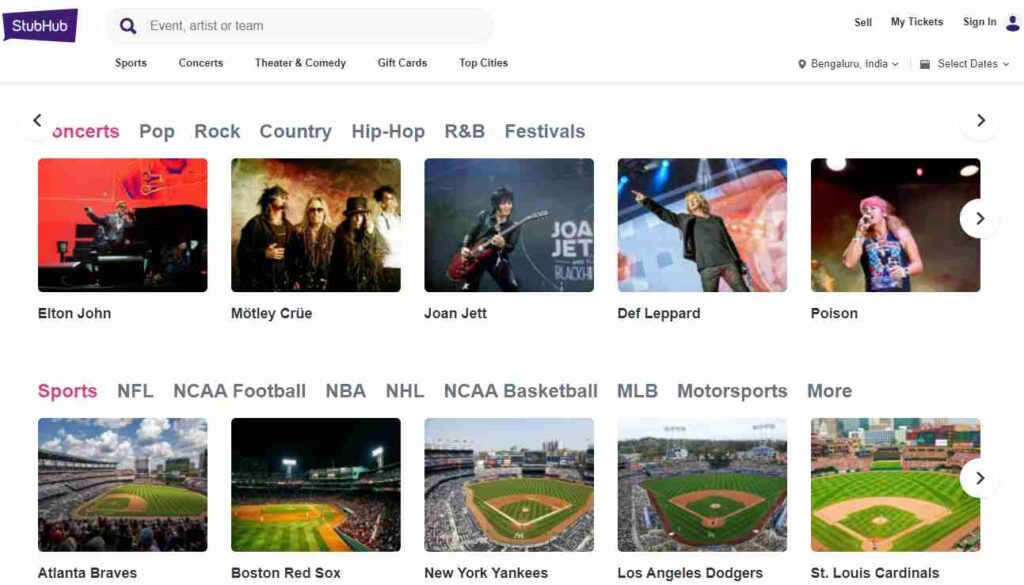This image showcases the homepage of the StubHub website. In the top left corner, a purple speech bubble logo prominently displays the word "StubHub" in white text. To the right of this logo, there is a search bar accompanied by a purple magnifying glass icon, inviting users to search for events, artists, or teams.

Directly below the search bar, are several navigation categories labeled: "Sports," "Concerts," "Theater & Comedy," "Gift Cards," and "Top Cities." In the top right corner, options for "Sell My Tickets" and "Sign In" are visible. Beneath these options, users can select their location, which is currently set to "Bengaluru, India," along with event dates for filtering search results.

The main content section begins with a focus on "Concerts," providing a detailed list organized by genres such as pop, rock, country, hip-hop, R&B, and festivals. Featured artists include Elton John, Mötley Crüe, Joan Jett, Def Leppard, and Poison, each accompanied by their respective images.

Adjacent to concerts, in the section labeled "Sports," users can explore events categorized under NFL, NCAA Football, NBA, NHL, NCAA Basketball, MLB, Motorsports, and more. A gallery of baseball team icons with images of their home fields includes the Atlanta Braves, Boston Red Sox, New York Yankees, Los Angeles Dodgers, and St. Louis Cardinals.

The detailed and organized layout ensures users can easily navigate and explore various entertainment and sporting events according to their preferences.